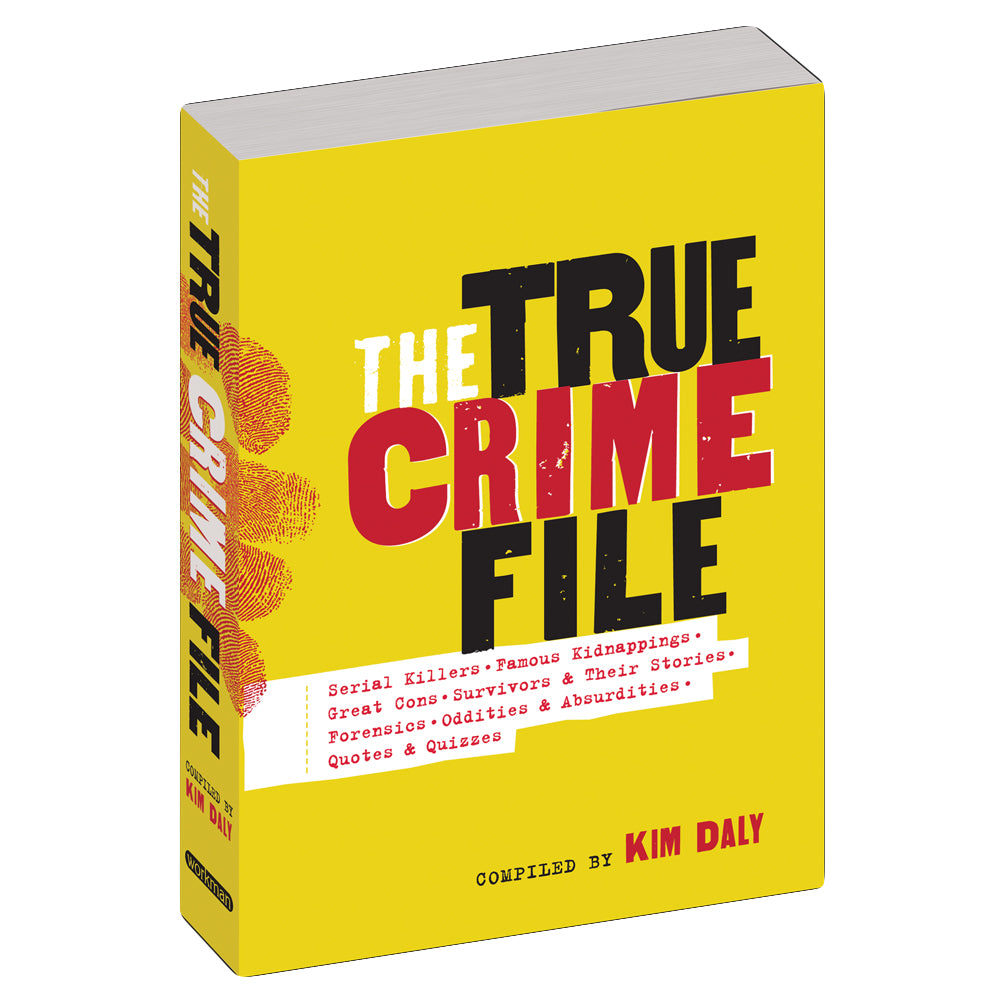This image features an upright, bright yellow paperback book titled "The True Crime File." The title is prominently displayed in white, black, and red font. Beneath the title, a white bar spans the cover with red text listing the contents: "Serial Killers, Famous Kidnappings, Great Cons, Survivors and Their Stories, Forensics, Oddities, and Absurdities, Quotes, and Quizzes." The book is compiled by Kim Daly, as indicated in black and red text at the bottom of the cover. A distinctive bloody handprint stretches across the spine and wraps around to the front, adding a dramatic touch. The spine also features the title "The True Crime File" in black and white text. The background of the image is pure white, accentuating the book's vivid yellow cover.